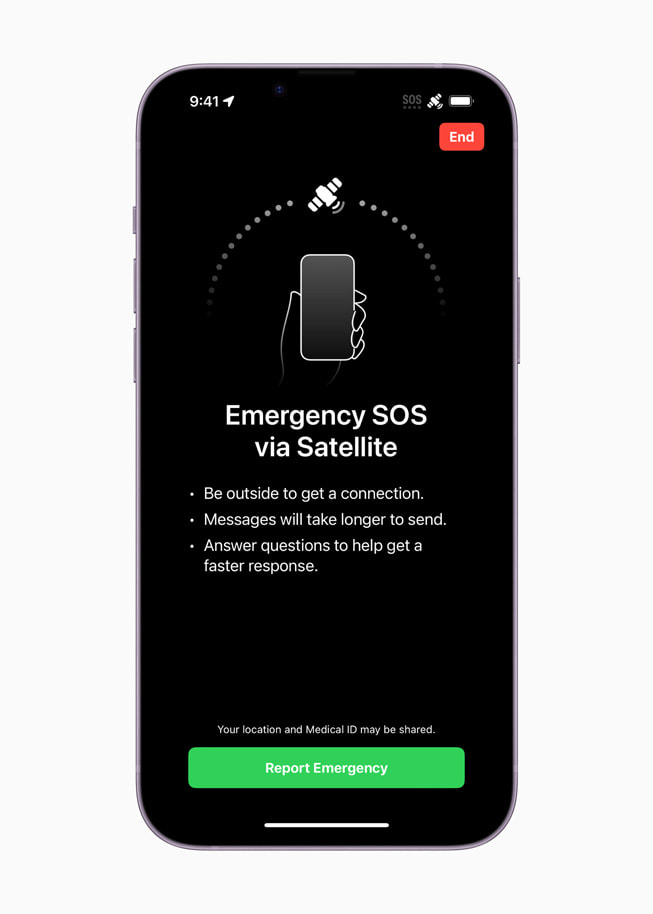The image displays a traditional Apple-style smartphone centered against an off-white background. The phone features a black screen with the time 9:41 in the upper left corner. On the right side, the battery percentage is shown, and below it, in a red square, the word "End" is displayed. 

On the screen, an important message is presented with a digital hand holding another cell phone. The text at the top reads "Emergency SOS via satellite." Below this are three bullet points in white text: "Be outside to get a connection," "Messages will take longer to send," and "Answer questions to help get a faster response." At the bottom of the screen, a green rectangular banner states "Report Emergency" in white text. Just above this green banner, there's a notice indicating that "Your location and medical ID may be shared."